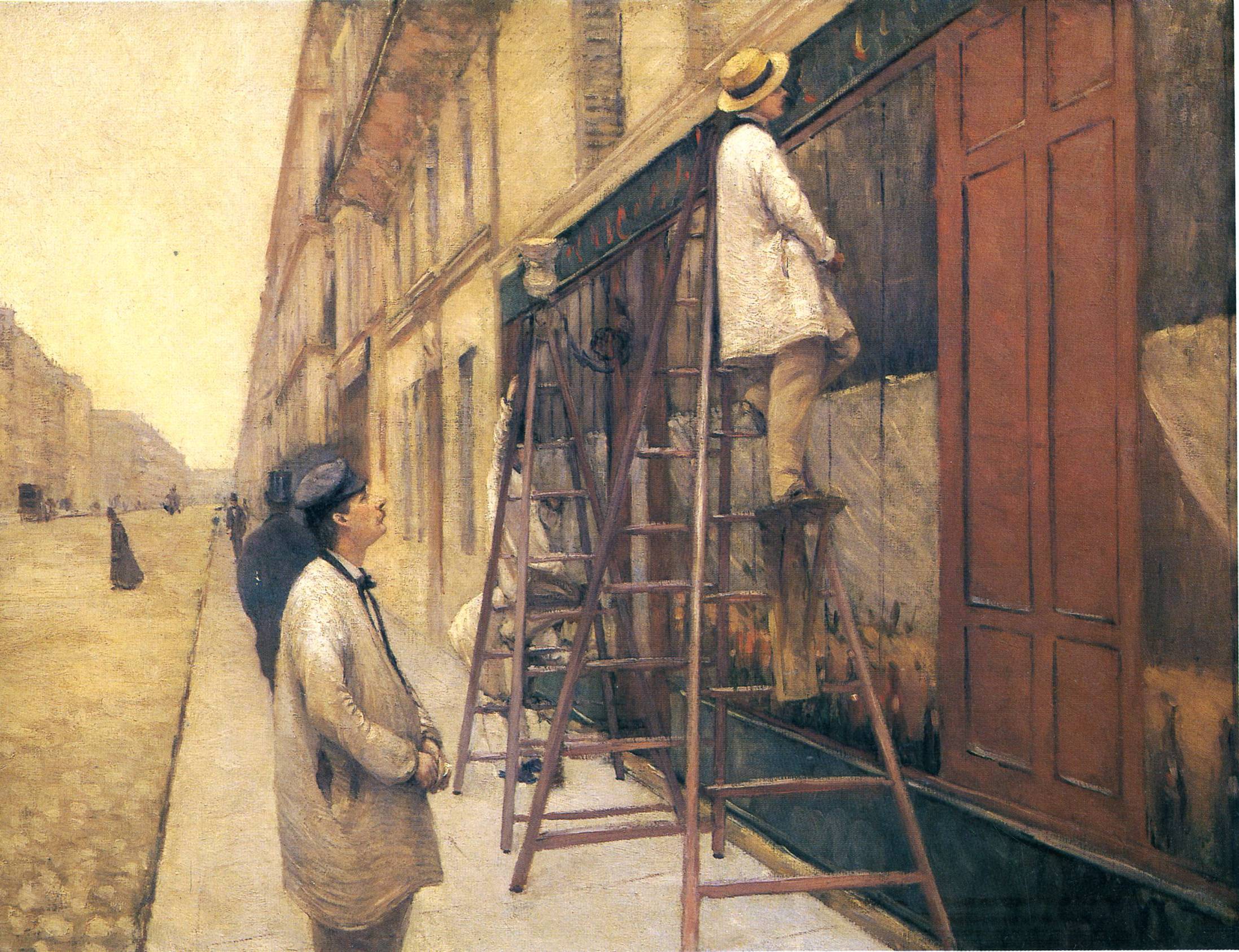The image is a highly detailed painting, likely from the 19th or early 20th century, depicting a street scene in warm, muted earthy tones. Central to the composition, on a sidewalk fronting a building, there are several men engaged in some form of work involving ladders. One man in tan pants and a long white jacket, topped with a straw boater hat, stands on the first ladder, facing a large brown wooden door set against a black wall. Behind him on a second ladder is another man, whose activities are less discernible. Nearby on the sidewalk, a third man clad in a similar jacket and wearing a dark newsboy cap observes the scene. In the background, individuals in dark suits and top hats stroll the street, where horse-drawn carriages can also be seen. The storefront, featuring wooden doors and windows displaying bottles, adds to the historical ambiance. Overall, this scene captures a bustling outdoor moment, possibly in the middle of the day, reminiscent of artistic works you'd expect to find displayed in a museum.